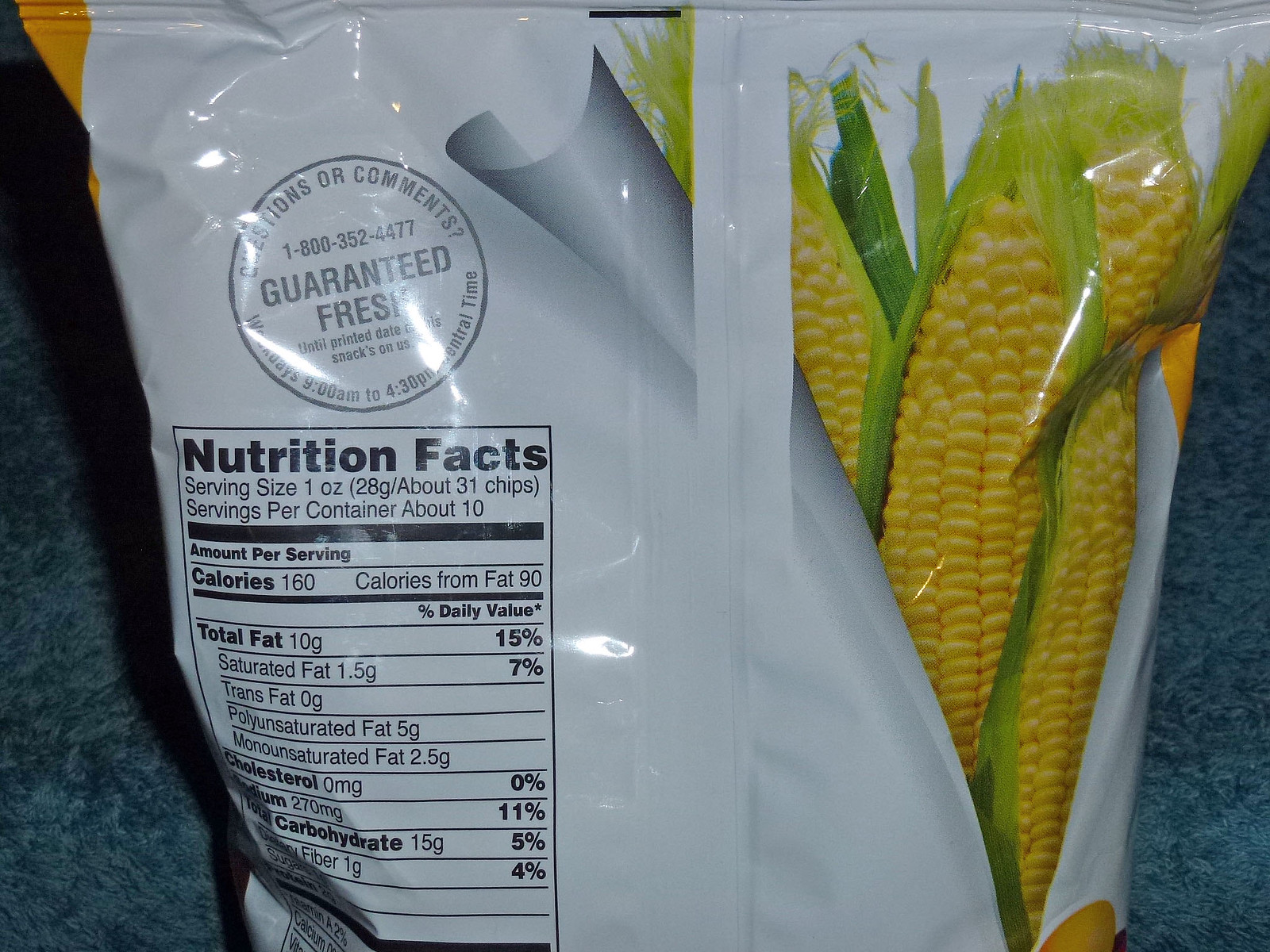The image is the backside of a package of corn-based chips. On the right side of the package, there is a color picture of three ears of yellow corn, partially husked with green husks still attached. The left side features the nutritional facts on a white label. The details include: serving size 1 ounce (28 grams), approximately 31 chips per serving, and about 10 servings per container. Per serving, it lists 160 calories, with 90 calories from fat, 10 grams of total fat (15%), 1.5 grams of saturated fat (7%), 5 grams of polyunsaturated fat, 2.5 grams of monounsaturated fat, 0 milligrams of cholesterol, 270 milligrams of sodium, 15 grams of total carbohydrates, and 1 gram of dietary fiber. There is also a stamp above the nutritional facts that reads "guaranteed fresh." The package is set against a background that appears to be a white and blue felt tablecloth, carpet, or blanket.